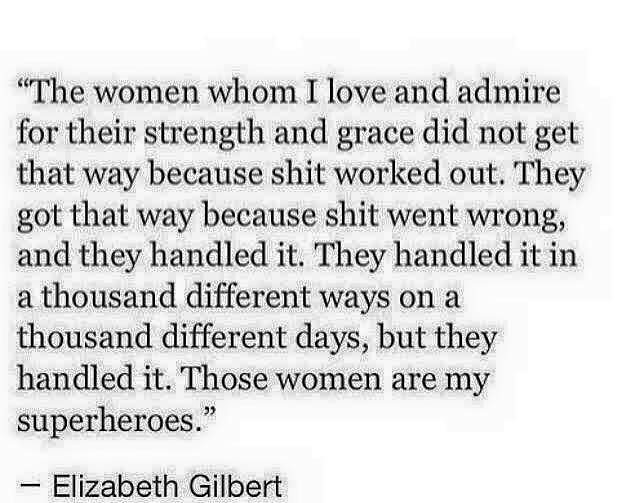The image features a quote by Elizabeth Gilbert, displayed in black text on a white background. The quote reads: "The women whom I love and admire for their strength and grace did not get that way because shit worked out. They got that way because shit went wrong and they handled it. They handled it in a thousand different ways on a thousand different days, but they handled it. These women are my superheroes." The text is left-aligned and takes up most of the frame, rendered in what appears to be a Times New Roman font, except for "Elizabeth Gilbert" at the bottom, which is in a sans-serif font like Calibri or Arial. Additionally, the text has a light blue shadow, creating a slightly grainy and dizzying effect around the letters.